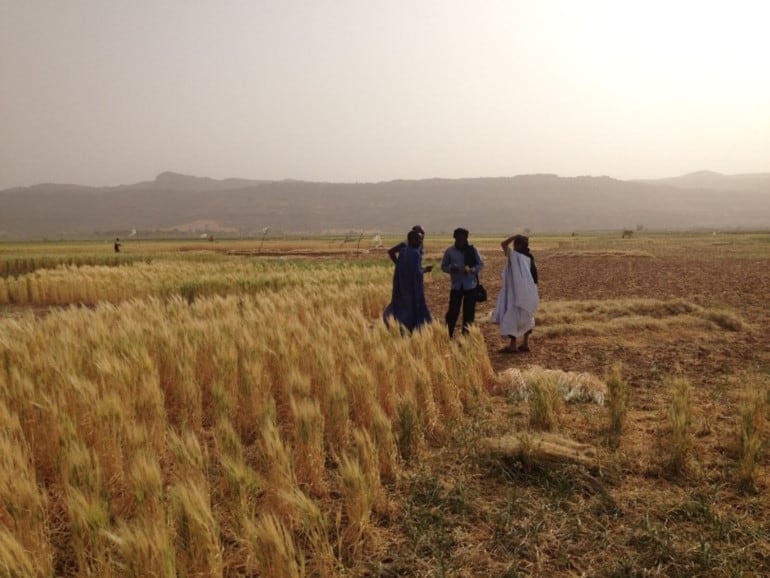In this photograph, taken in a vast outdoor field that could possibly be in Africa, we see a mix of cut and uncut wheat. The uncut crop is mostly brown, stretching out toward the left side of the image, while the right side of the field is empty where the wheat has already been harvested. The scene is somewhat obscured by blurriness and smoke in the air, making the sky appear mostly white with a bright spot in the top right corner. 

Three to four dark-skinned individuals, including women in long dresses, stand in the middle of the field, engaged in conversation and appearing to organize the harvested bundles of wheat. They are surrounded by the expansive field with more crops visible toward the back left. The background features hazy hills or mountains, adding a sense of grandeur to the setting. Despite the challenging, dry, and hot conditions, the people’s diligent work in harvesting the wheat is clearly evident, and the neatly bundled crops attest to their dedicated efforts.